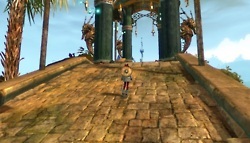A small, rectangular, landscape-oriented photograph captures a stone ramp ascending toward a columned edifice. The structure, adorned with four large, dark columns supporting an arched or vaulted roof, is partially cropped at the top of the image. A vivid blue sky filled with scattered clouds serves as a picturesque backdrop, complemented by the presence of palm trees along the ramp's side. A person is seen ascending the ramp, identifiable by the wide-brimmed hat hanging down their back and their distinctive red leggings paired with a jacket. Additionally, some intricate metalwork can be observed near the edifice. The stone surface of the ramp is a light brown hue, contrasting with the dark columns and vibrant sky.